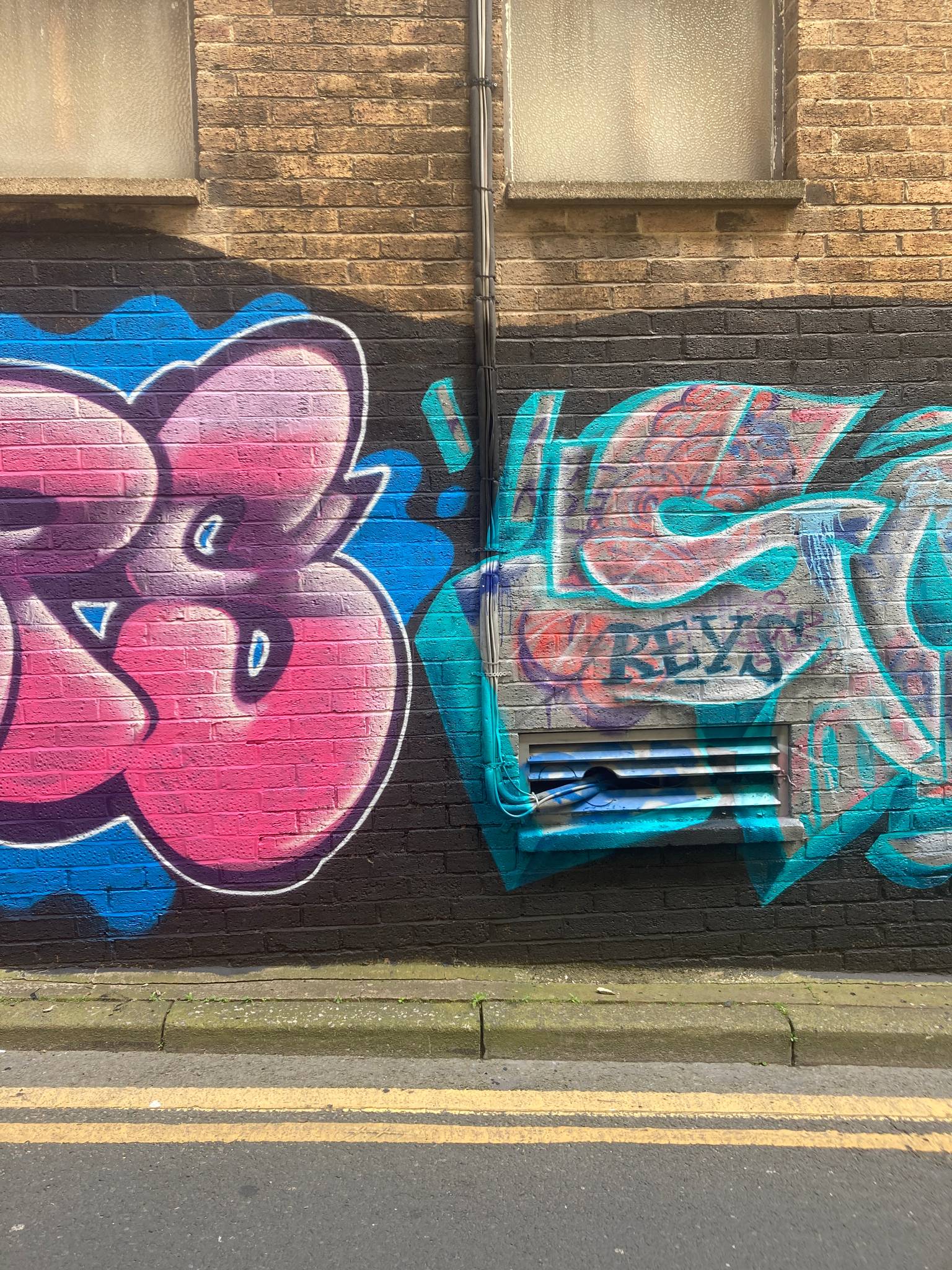The photograph captures a street scene featuring a tan-brick building adorned with vibrant graffiti. Dominating the foreground are two solid yellow lines marking the center of the asphalt street, which runs alongside a narrow sidewalk. This sidewalk abuts the building, whose brick exterior transitions from its natural brownish hues at the top to a graffiti-covered section below.

At the upper portion of the building, two windows are partially visible, situated just above a layer of black spray paint that serves as a backdrop for the graffiti. Descending from one of these windows are coiled wires leading to a vent, both of which have been spray-painted. The graffiti predominantly features layers of blue and pink paint. On the left side, there is a blue splotch and large, partially obscured pink and black letters, including an "R" and an "S." Below, the artwork showcases additional letters in turquoise, gray, and green tones, including the word "RAYS" (spelled out as R-E-Y-S) in vivid blue. Amidst the colorful chaos, a red heart can be seen, adding to the intricate tapestry of urban art.